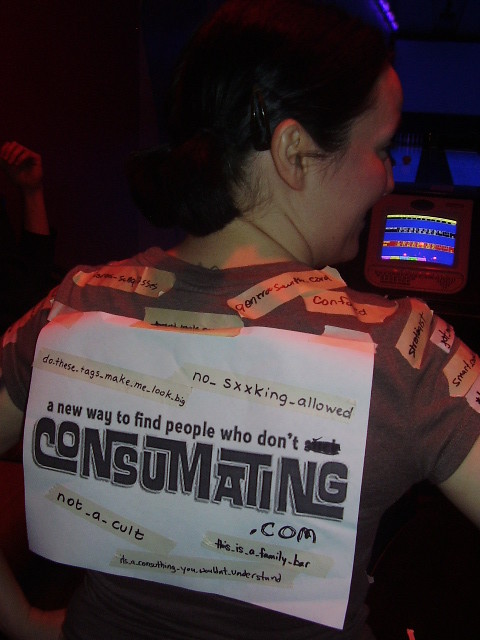The image depicts the back of a Caucasian woman with short dark brown hair tied in a small ponytail, secured by a dark red (burgundy) hair tie, and accessorized with a black clip behind her ear. She is wearing a brown short-sleeved t-shirt, and the scene is set in a dark indoor environment, with a lit computer screen visible in the distance. Covering her back are numerous pieces of painter's tape with messages written in black marker, and a white printed sign. The tape messages collectively read phrases like, "no_sxxking_allowed" and "do.these.tags.make.me.look.big." The central white sign on her back prominently states, "A new way to find people who don't suck—consummating.com" with the word "suck" struck through and replaced with "consummating." Additional tape messages include statements like "not_a_cult," "this_is_a_family_bar," and an indistinct message that appears as "RLS_a_consulting_you_something_want_understand." The woman's surroundings are dark, especially in the upper left corner, which is almost pitch black, and the image is tall and narrow, focusing closely on the details of her back and the displayed messages.